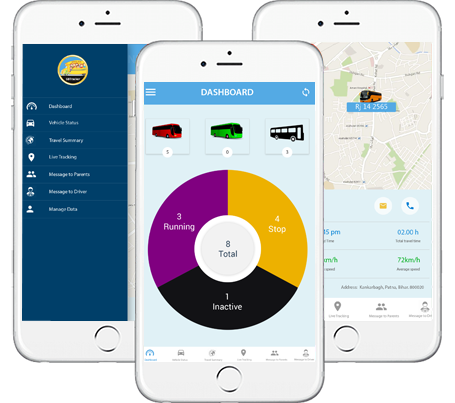The image depicts a square composition with a white background that blends seamlessly with the image's edges, making them indistinguishable. At the forefront are three smartphones, arranged in a triangular formation. The central phone is positioned slightly lower than the two flanking it, creating a descending diagonal line.

Each phone has a slightly off-white hue and features a single button at the bottom, reminiscent of an iPhone design. The screens display different interfaces:

1. **Left Phone:** This phone screen showcases a dark blue navigation pane with seven options. The text on these options is too small to decipher.

2. **Center Phone:** This screen presents a clean interface featuring a pie chart, depicted in various colors representing different segments.

3. **Right Phone:** The display indicates a map view from a bird's-eye perspective. The map includes various roads and green areas, indicating parks or other vegetated spaces, along with direction indicators at the bottom.

Overall, the image captures technological devices with distinct functionalities, positioned thoughtfully to create a visually balanced layout.